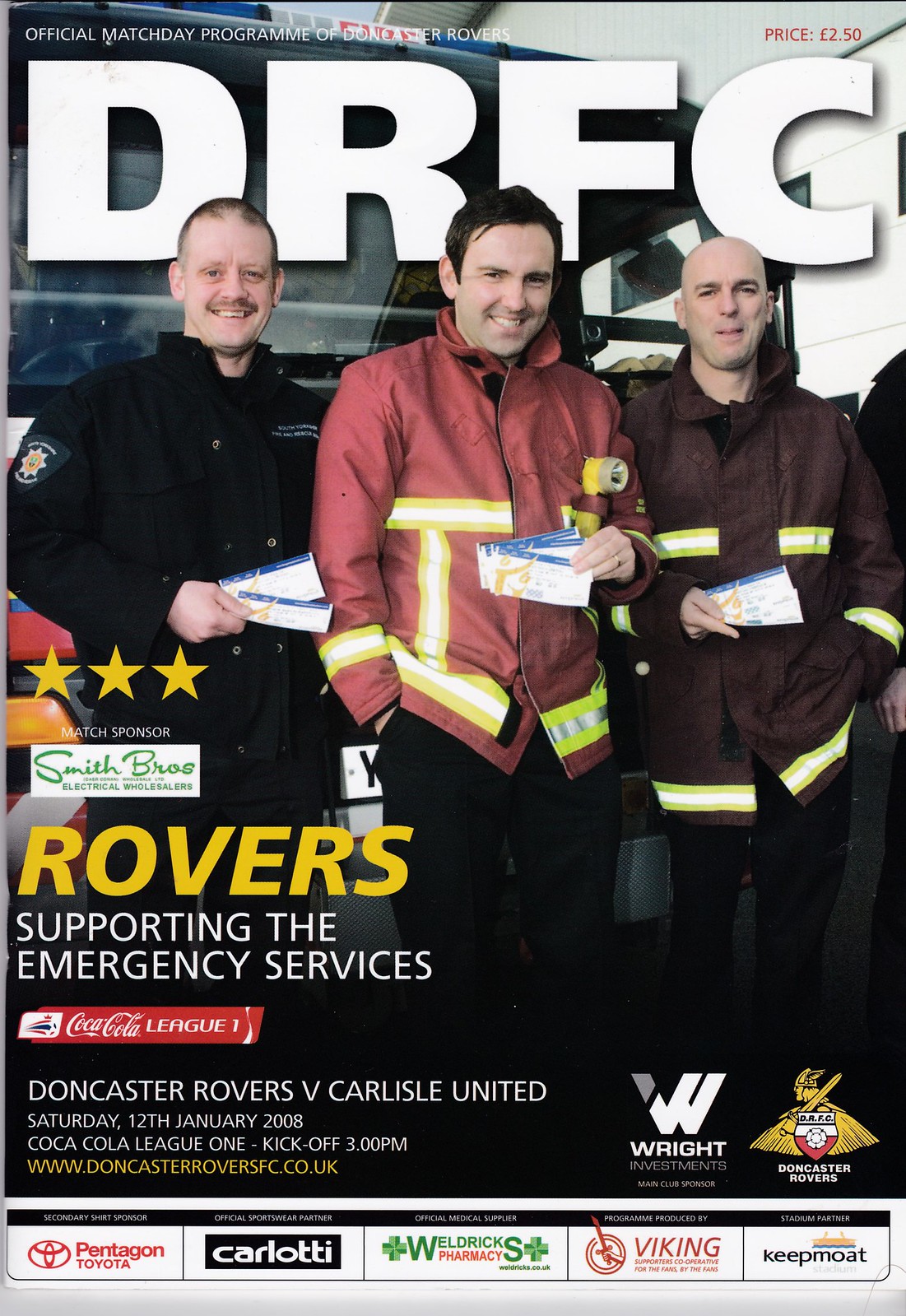The front cover of the Official Match Day Program for Doncaster Rovers, priced at $2.50, prominently features the team acronym "DRFC" in big, bold white letters at the top. Just above this, smaller white text reads "Official Match Day Programme for Doncaster Rovers." Below, the title "Rovers" in large yellow letters leads to the subtitle "Supporting the Emergency Services," sponsored by Coca-Cola. This edition covers the match between Doncaster Rovers and Carlisle United on Saturday, January 12, 2008, with a Coca-Cola League One kickoff at 3 p.m.

Central to the design is an image of three gentlemen standing in front of a large bus, each showcasing emergency service gear. The first man on the left, who is balding with a moustache, wears a dark black jacket and holds two tickets. The middle man has mid-length brown hair, dons a red jacket with visible fluorescent accents, and holds one ticket. The third man, also bald, wears a burgundy jacket with fluorescent strips and another ticket. Various advertisements, including one for Coca-Cola and another from "Match Sponsor Smith Bros Electrical," line the bottom, along with the team's website, www.doncasterroversfc.co.uk.